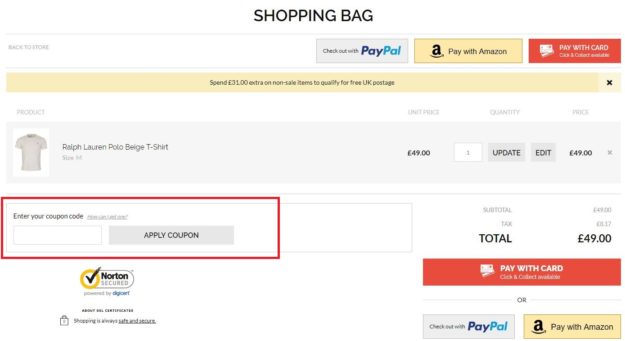**Screenshot of a Shopping Bag Checkout Screen**

The screenshot captures the checkout interface of an online shopping website. At the top center of the screen, it prominently displays the heading "Shopping Bag." Below this heading, three payment options are available, each within a clickable rectangle: "Checkout with PayPal" in a gray rectangle, "Pay with Amazon" in a yellowish rectangle, and "Pay with Card" in an orange-red rectangle.

A prompt beneath these options informs users that spending £31 more on non-sale items will qualify them for free UK postage. Following this message, details of the current item in the shopping cart are presented: a beige Ralph Lauren polo t-shirt. Although the size is mentioned, the font is too small to be legible. To the left of the product details is a photo of the t-shirt. The price details indicate that the unit price of the t-shirt is £49, the quantity is 1, and the total price is £49.

Directly below the t-shirt photo, there's a section inviting users to enter a coupon code. This section includes an empty text box for the code entry and a gray rectangle labeled "Apply Coupon." The entire coupon code entry area is outlined with a red rectangle.

Further below, the security assurance symbol "Norton Secured," sponsored by DigiCert, is displayed alongside the message "Shipping is always safe and secure."

In the bottom right section of the screen, the order summary is shown. It lists the subtotal as £49. Although the tax amount is mentioned, here again, the font is too small to be read. The total amount due is confirmed as £49. Users are given the option to finalize the purchase by clicking "Pay with Card" in a red rectangle or choose alternate payment methods via PayPal or Amazon.